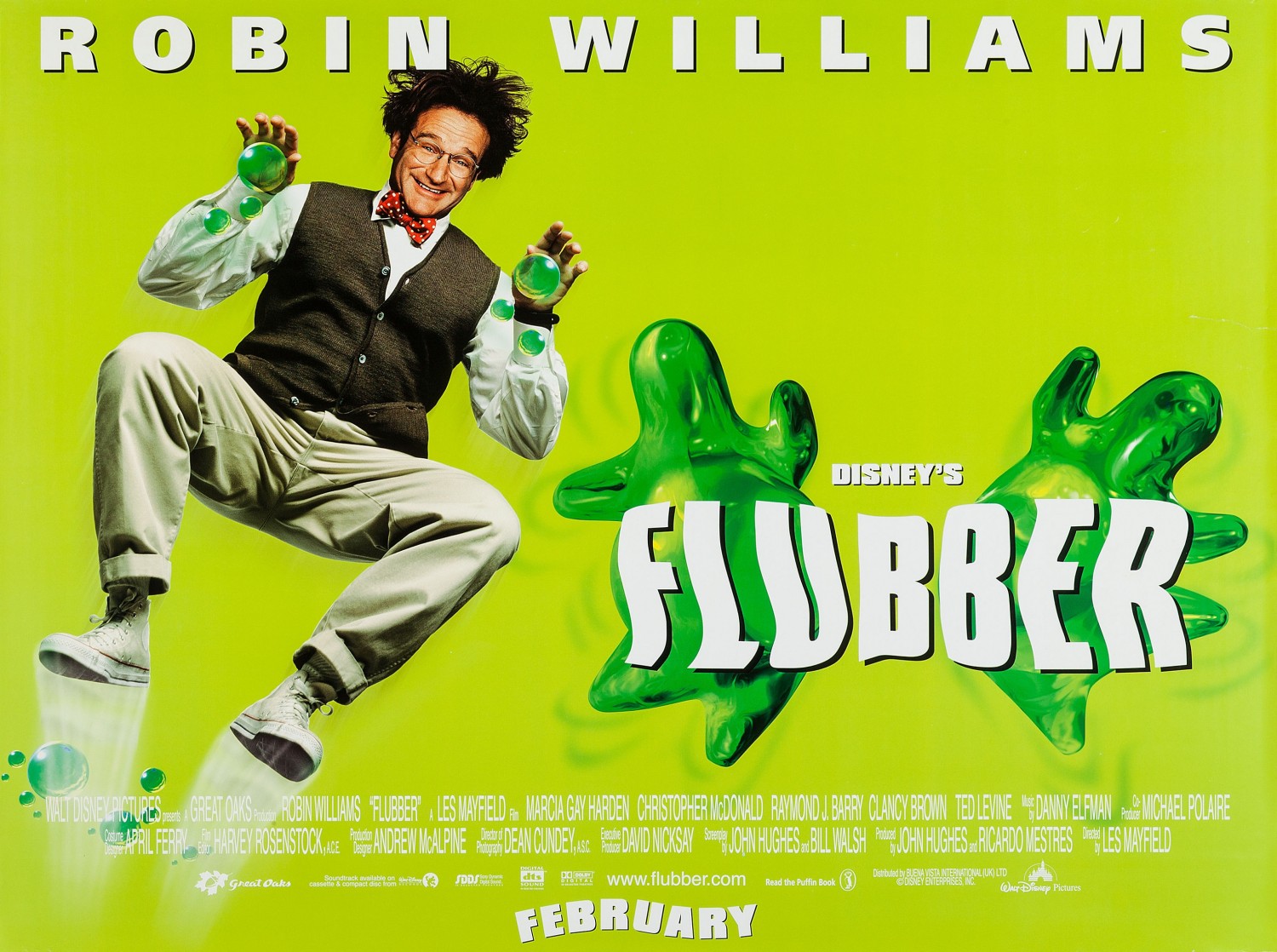The advertisement is a vibrant movie poster for Disney's "Flubber" featuring Robin Williams. The background is a striking lime green, and at the top, bold white block letters spell out "Robin Williams," with slight spacing between each letter. Positioned on the left side, Robin Williams is captured in an energetic pose, jumping with his knees slightly bent and arms raised, as if bouncing. His hair appears disheveled as if he's just leaped off a trampoline. He is wearing a white button-up shirt, a brown vest, tan pants, and a red plaid bowtie. Clutched in his palms and also floating nearby are bright green, animated blobs of the titular flubber, depicted with wavy lines to suggest motion. Engaging and whimsical, the poster’s right side showcases the text "Disney's Flubber" in a playful font, with "Disney's" in smaller letters and "Flubber" in larger, wavy capital letters. Beneath this, additional movie credits are listed, culminating at the bottom of the poster with the release timeframe marked in similar wavy capital letters: "February."